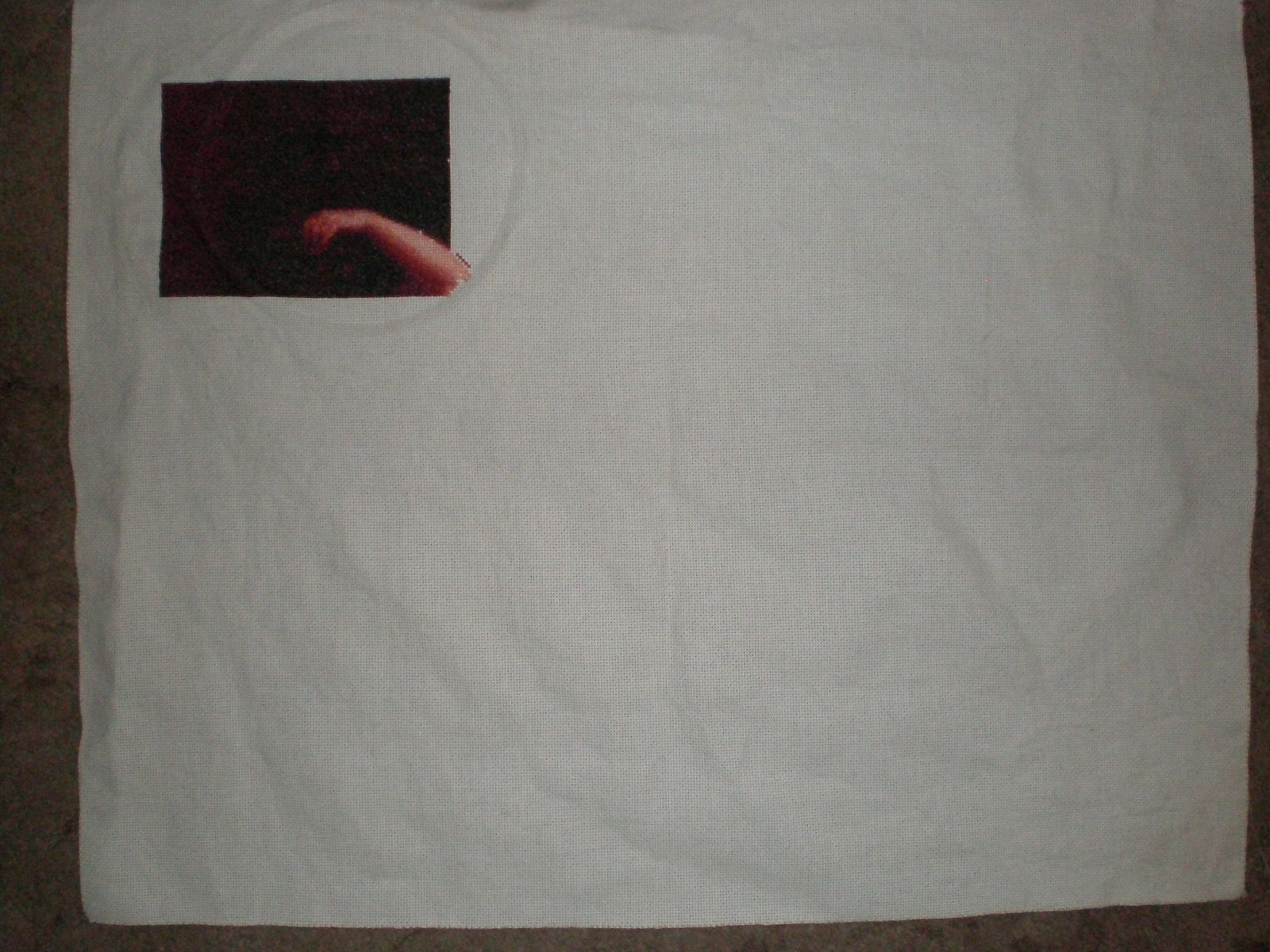This photograph features a highly crumpled piece of paper, or possibly a similarly textured white fabric, lying flat on a surface that appears to be dark grey, perhaps black. The overall lighting is dim, giving the image a muted appearance. The object in question is predominantly white and rectangular, positioned horizontally. In the top left-hand corner of the frame, there's a solid black box. Meanwhile, in the bottom right-hand corner, an arm extends into the shot, cut off around the elbow area. The arm, aligned with the corner, introduces an organic element to the otherwise static composition. The forearm and hand, pale in color, rest upon the wrinkled white surface, creating a stark contrast against the dark background.